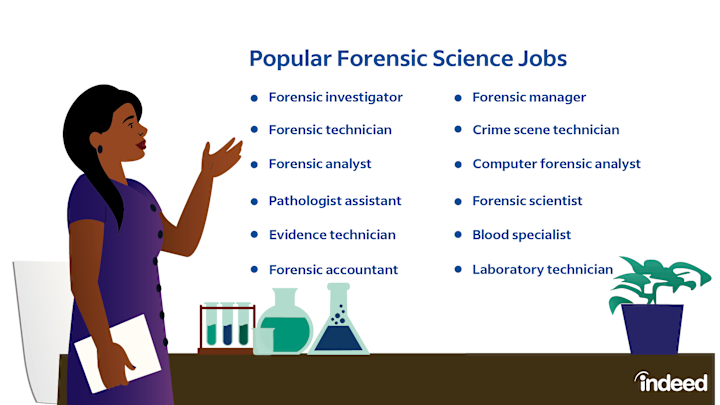The infographic, set against a white background with blue text, is titled "Popular Forensic Science Jobs." It features a comprehensive list of twelve job titles arranged in two columns of six. On the left, the jobs include: Forensic Investigator, Forensic Technician, Forensic Analyst, Pathologist Assistant, Evidence Technician, and Forensic Accountant. On the right, the list further includes: Forensic Manager, Crime Scene Technician, Computer Forensic Analyst, Forensic Scientist, Blood Specialist, and Laboratory Technician.

To the left of this text, there is a digitally illustrated woman depicted with a purple dress and black hair. She holds a white notepad in her right hand and extends her left hand towards the job titles, seemingly introducing them. Behind the woman is a white chair and a brown table adorned with scientific props such as round-bottomed flasks, an Erlenmeyer flask, and test tubes, indicating a chemistry setting. A blue potted plant with green leaves is positioned on the right side of the table. At the bottom right corner of the infographic, the Indeed logo appears in white text.